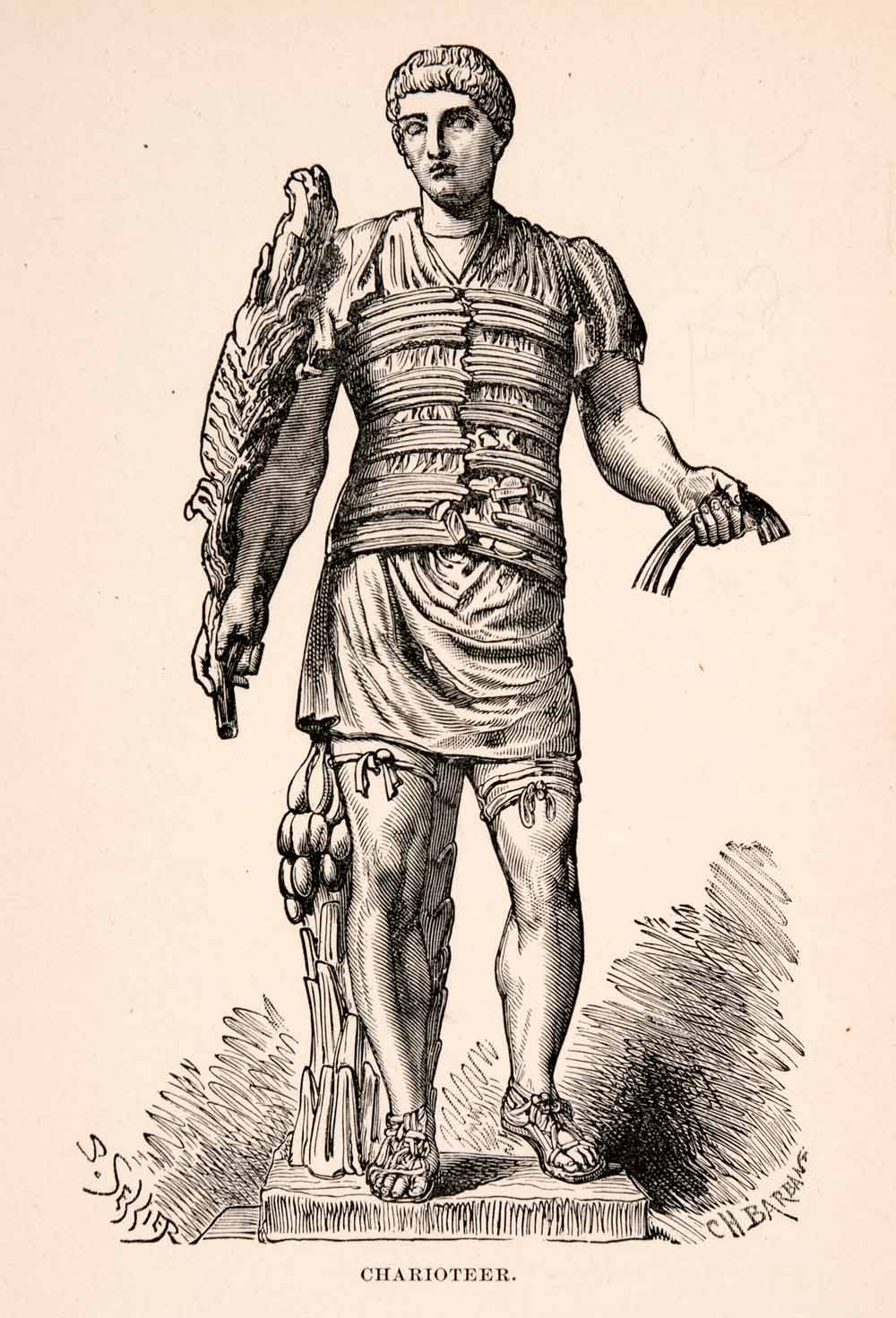This is a black-and-white engraving on a pale pink background, depicting what appears to be a Roman man or soldier. The figure stands facing forward on a short stone pedestal or platform that casts shadows beneath it. The man has a Caesar-like short haircut and his eyes are carved without pupils, suggesting a statue-like quality. Clad in a mid-thigh-length tunic with gladiator-style elements, he has straps tied around his upper thighs and across his waist. His feet are shod in sandals. He holds a large feather that extends to his shoulder in his right hand, while his left hand presents a piece of cloth. Detailed shading work adds depth, particularly at the base of the platform. Below the drawing, the word "charioteer" is inscribed. In the lower right corner, there's a signature by the artist, C.H. Barbain, and the name S. Sellier is noted in the left corner.